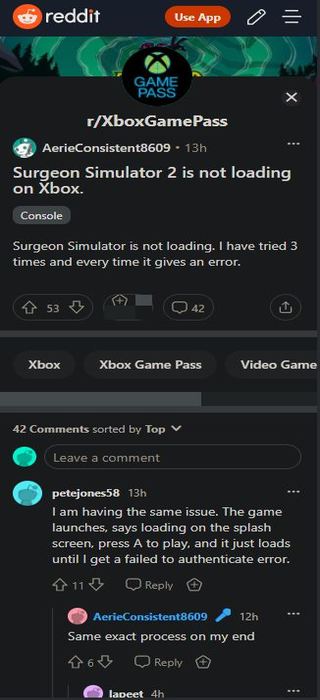The screenshot showcases a Reddit page viewed on a computer screen with a black background. At the top, the word "reddit" is displayed in white text, accompanied by a red circle featuring an illustration of a white alien face. Adjacent to this, there is a red button with the text "Use App" in white, next to a white pencil icon.

Below this header section, a light green banner depicts a scene with trees, the sky, and varying shades of green foliage. Centered within this banner is a black circular logo with the text "Game Pass" in white. Beneath it, the subreddit name "r/XboxGamePass" is prominently displayed, followed by the username "aerieConsistent8609" and the timestamp "13h".

The post titled "Surgeon Simulator 2 is not loading on Xbox" is clearly outlined. It includes the tags "Console" and reads "Surgeon Simulator is not loading. I've tried three times and every time it gives me an error. The error number is 53." 

Scrolling down, you see "Xbox" in white text, followed by "Xbox Game Pass" and "Video Game" also in white. A gray horizontal line separates the post from the comment section, which shows "42 comments sorted by top". 

A blue circle marks the prompt "Leave a Comment," and the first comment is by user "PeteJones58", stating: "I'm having the same issue. The game launches, says loading on the splash screen, press A to play, and it just loads until I get a failed to authenticate error."